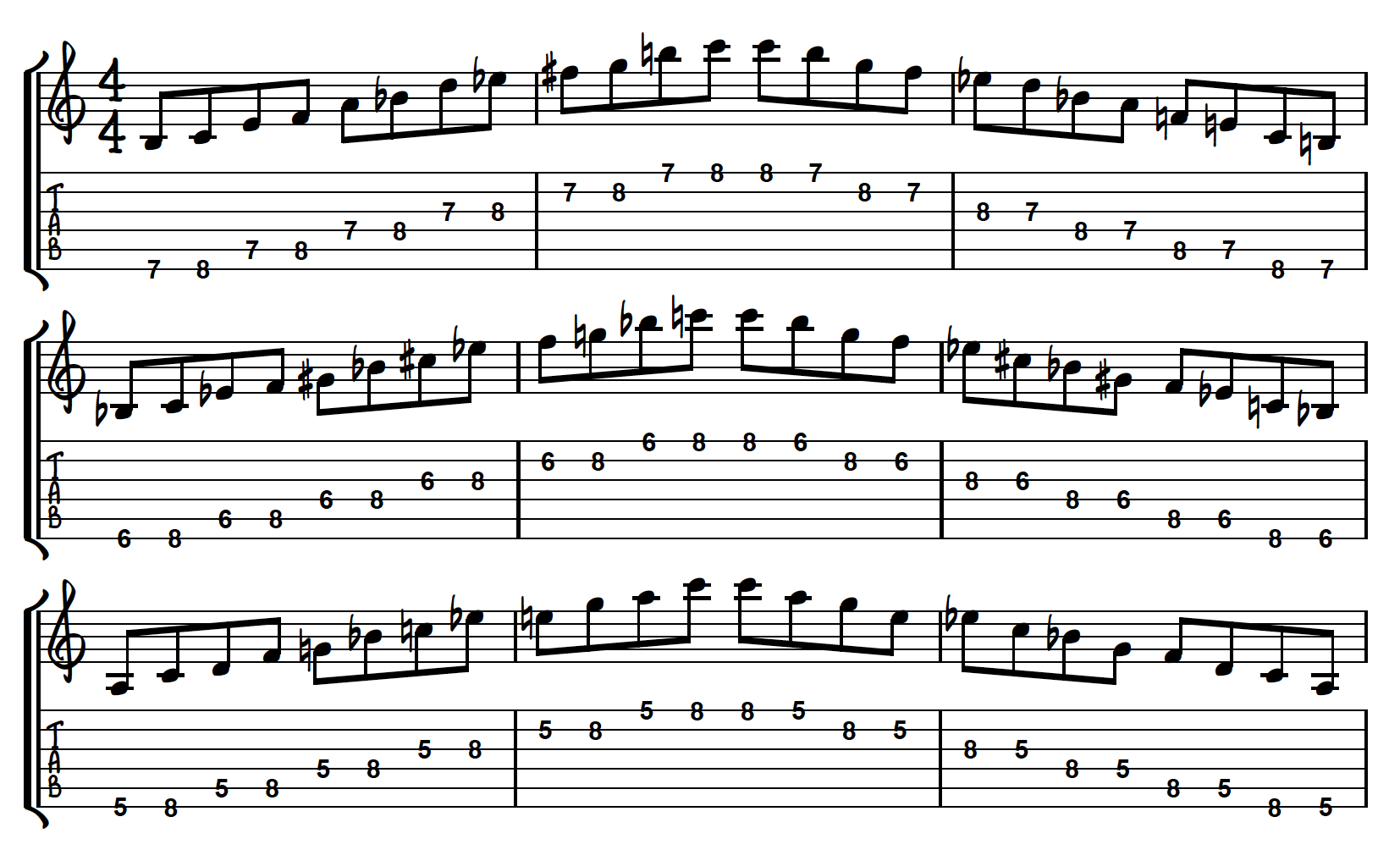The image depicts a detailed sheet of music with three distinct staffs, each containing notes accompanied by numerical values. The top staff features a time signature of 4/4 and includes a pattern of notes marked with corresponding numbers, primarily seven and eight, with some notes designated as sharp or flat. The middle staff's notes are paired with numbers ranging from six to eight, showing a recurring sequence. Similarly, the bottom staff displays a number sequence from five to eight. Each staff has notes positioned within rectangles on horizontal lines, indicating their pitch, possibly useful for learners of piano or guitar. The numerical values associated with the notes form a visual pattern that rises and falls, creating a hill-like structure across the staff lines. The image's background is predominantly white, with the music in black, providing a clear visual contrast for easy reading and interpretation.